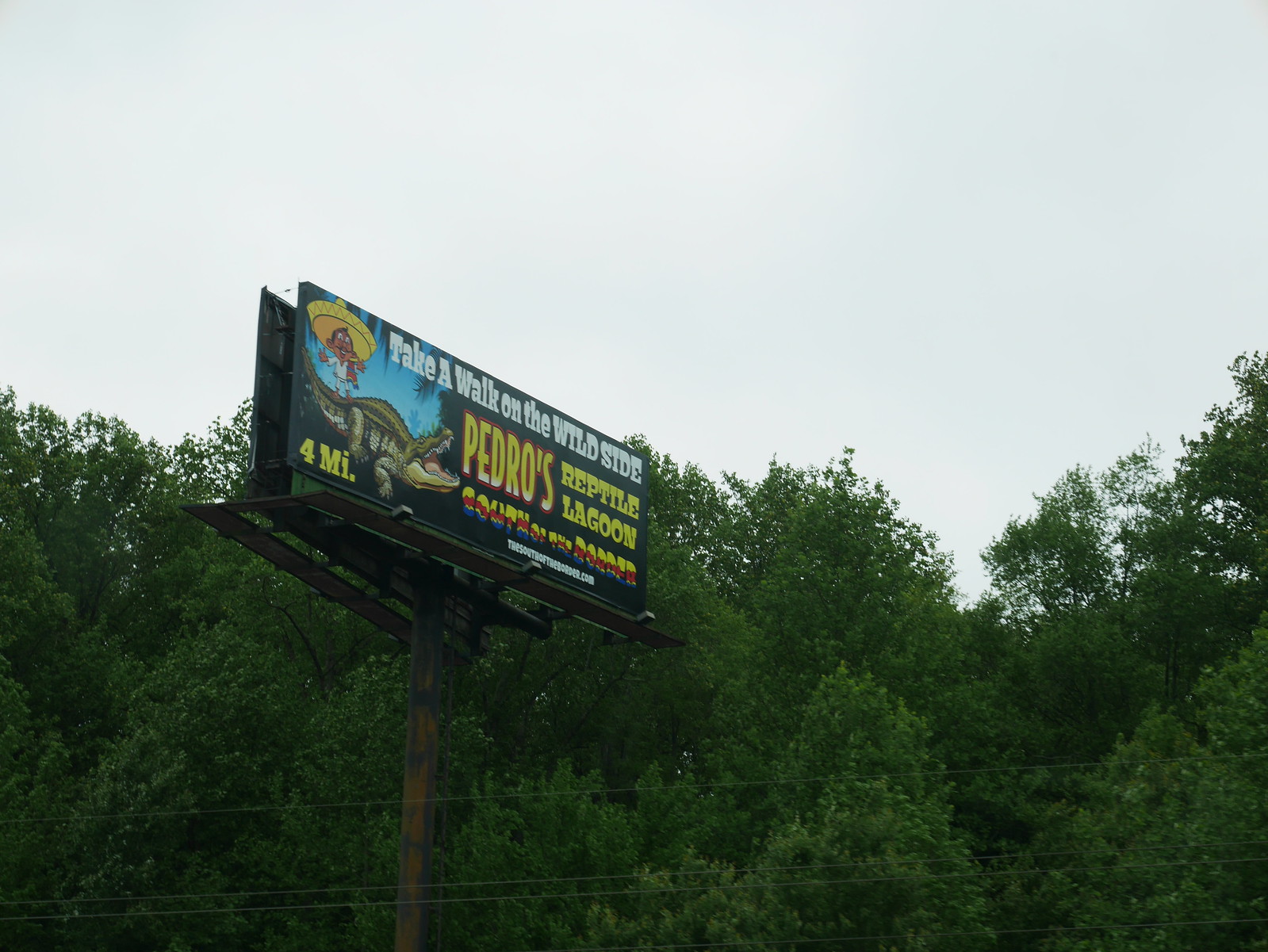The image depicts a vintage billboard situated against a lush, green backdrop of trees, suggesting a forested area along the side of a freeway. At the bottom of the image, several cable wires are visible, running horizontally. The billboard is mounted on an old wooden stand, contributing to its rustic appearance. The advertisement on the billboard features a colorful illustration of a crocodile alongside a cartoonish Mexican man wearing a sombrero, a vibrant scarf, and a mustache. 

The text on the billboard is as follows:
- At the top, in bold white font: "Take a walk on the wild side."
- Below, in bright yellow font: "Pedro's Reptile Lagoon."
- Further down, in a tri-colored font: "South of the Border."
- At the bottom, a link reads: "Go to southoftheborder.com to learn more."
- In the bottom left corner, it indicates the distance to the destination: "4 miles."

The combination of vivid imagery and enticing text aims to lure passing travelers to the nearby attraction.